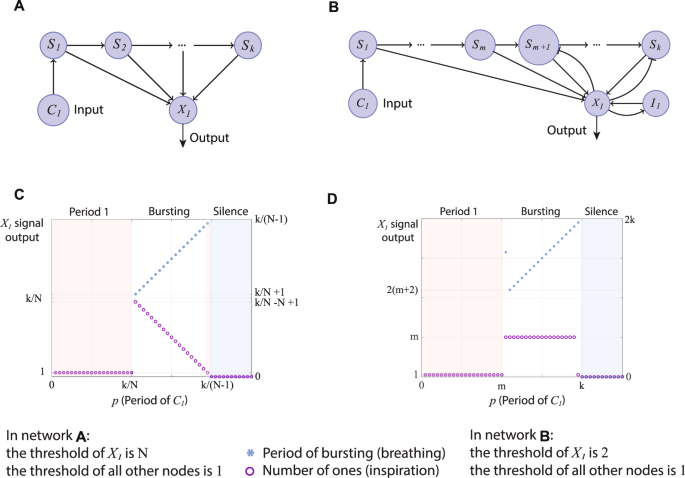The image displays a detailed diagram divided into four quadrants, labeled A through D. Quadrant A, located in the top left, features a diagram with five circular nodes labeled S1, S2, C1 (input), X1 (output), and SK, all with arrows pointing to X1. Quadrant B, to the top right, depicts a similar structure with seven circular nodes labeled for input and output, albeit in a different arrangement. 

In the bottom left, Quadrant C showcases a labeled diagram with terms such as X, signal output, KN, period 1, bursting, and silence. It is visually represented by a square shape containing a V-shaped line comprised of two colors: purple and blue. Quadrant D, at the bottom right, features a similar square diagram but includes three horizontal purple lines and a diagonal blue line, alongside the same labels as in C.

At the bottom of the page, text details the attributes of Network A and Network B. For Network A, it specifies that the threshold of X1 is N, while all other nodes have a threshold of 1. The text also mentions "period of bursting (breathing)" symbolized by a blue star, and "number of ones (inspiration)" represented by a purple circle with a white center. For Network B, the threshold of X1 is indicated as 2, with all other nodes maintaining a threshold of 1.